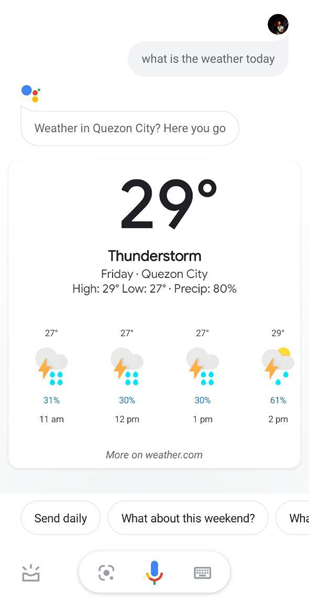This image depicts a weather app interface. On the right side, there's a blurry circular icon of a person, suggesting a user profile or an AI assistant prompt. The image prominently features the Google AI logo, consisting of a large blue circle, a small red circle, a slightly larger yellow circle, and a tiny green circle.

The weather forecast displayed is for Quezon City. The primary forecast reads "Weather in Quezon City: 29°C," with a thunderstorm predicted for Friday. Detailed hourly weather updates include:
- **11 a.m.:** 27°C, lightning and rain, 31% chance of precipitation.
- **12 p.m.:** 27°C, lightning and rain, 30% chance of precipitation.
- **1 p.m.:** 27°C, lightning and rain, 30% chance of precipitation.
- **2 p.m.:** 29°C, partially sunny with some rain, 61% chance of precipitation.

The forecast indicates consistent temperatures around 27°C with thunderstorms until 2 p.m., at which point the temperature rises to 29°C and the sun starts to appear. The app mentions "high 29°C, low 27°C, precipitation 80%."

At the bottom of the interface, there are several buttons, although some are partially cut off. One button indicates "More on weather.com," another prompts to "Send daily updates," and an additional cut-off button starts with "W-A," possibly a further feature or option related to weather updates.